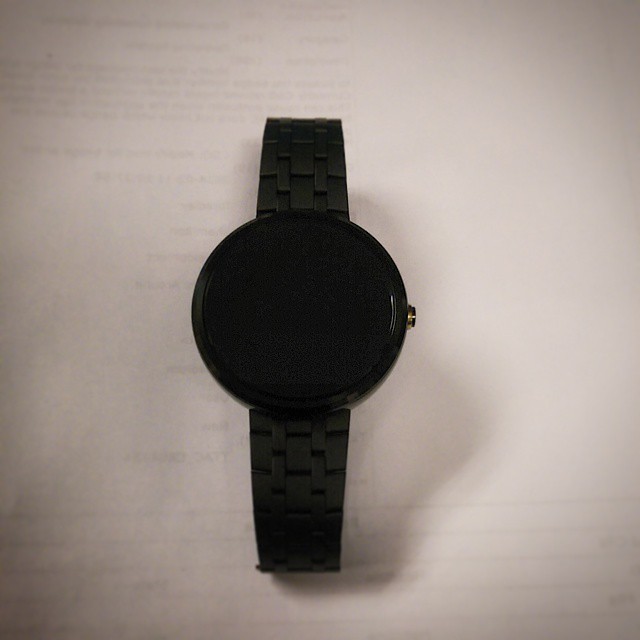The image depicts a black wristwatch with a completely dark, unlit screen, which appears to be glossy, possibly indicating it's a smartwatch. The watch features a dark silver dial on its right side. It rests on a white background, likely a piece of paper, beneath which faded black text is slightly visible. The wristband of the watch has a braided texture, giving it a distinctive look. The photograph is illuminated in such a way that a shadow is cast beneath the watch, emphasizing its three-dimensional form. No brand name or specific markings can be seen on the watch, making it difficult to identify its exact model or brand. The entire setup is against a beige-gray backdrop, contributing to the simple and focused presentation of the watch.